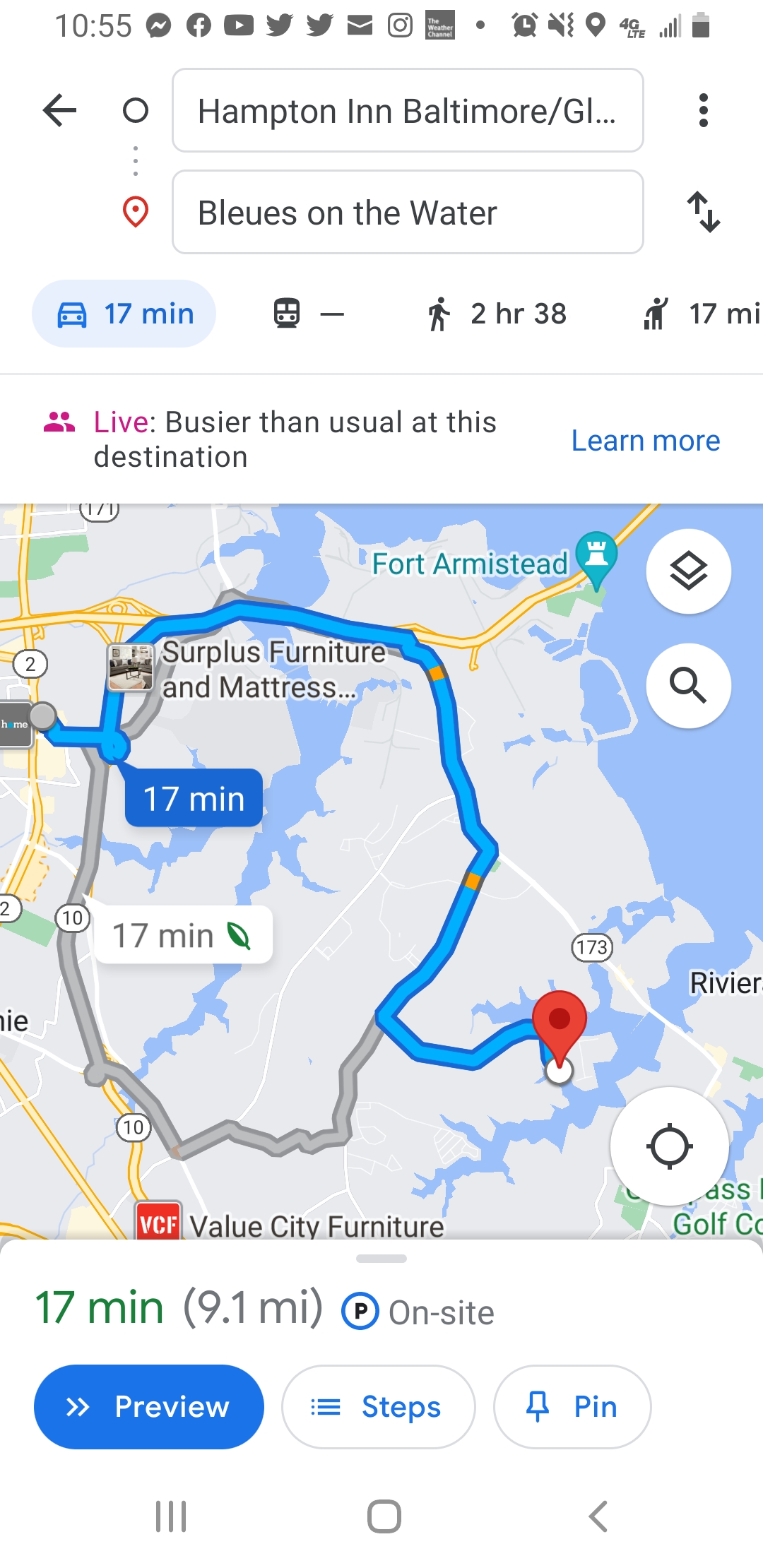This screenshot captures a Maps and Directions app on a mobile device without the phone itself being visible. The screen displays a navigation route from the Hampton Inn in Baltimore to a destination called Blues on the Water, estimated to be a 17-minute drive covering a distance of 9.1 miles, or a 2-hour and 38-minute walk. The route is highlighted in blue with an alternate path in gray, showcasing the journey around Fort Armistead and notable landmarks such as a surplus furniture and mattress store. The map also indicates the bay’s coastline, emphasizing the water along the route. Additionally, the app notes that the destination is busier than usual and mentions on-site parking. Notification icons for various apps like email, Twitter, YouTube, and Facebook are visible at the top of the screenshot, and standard navigation icons of home, back, and menu are positioned at the bottom.